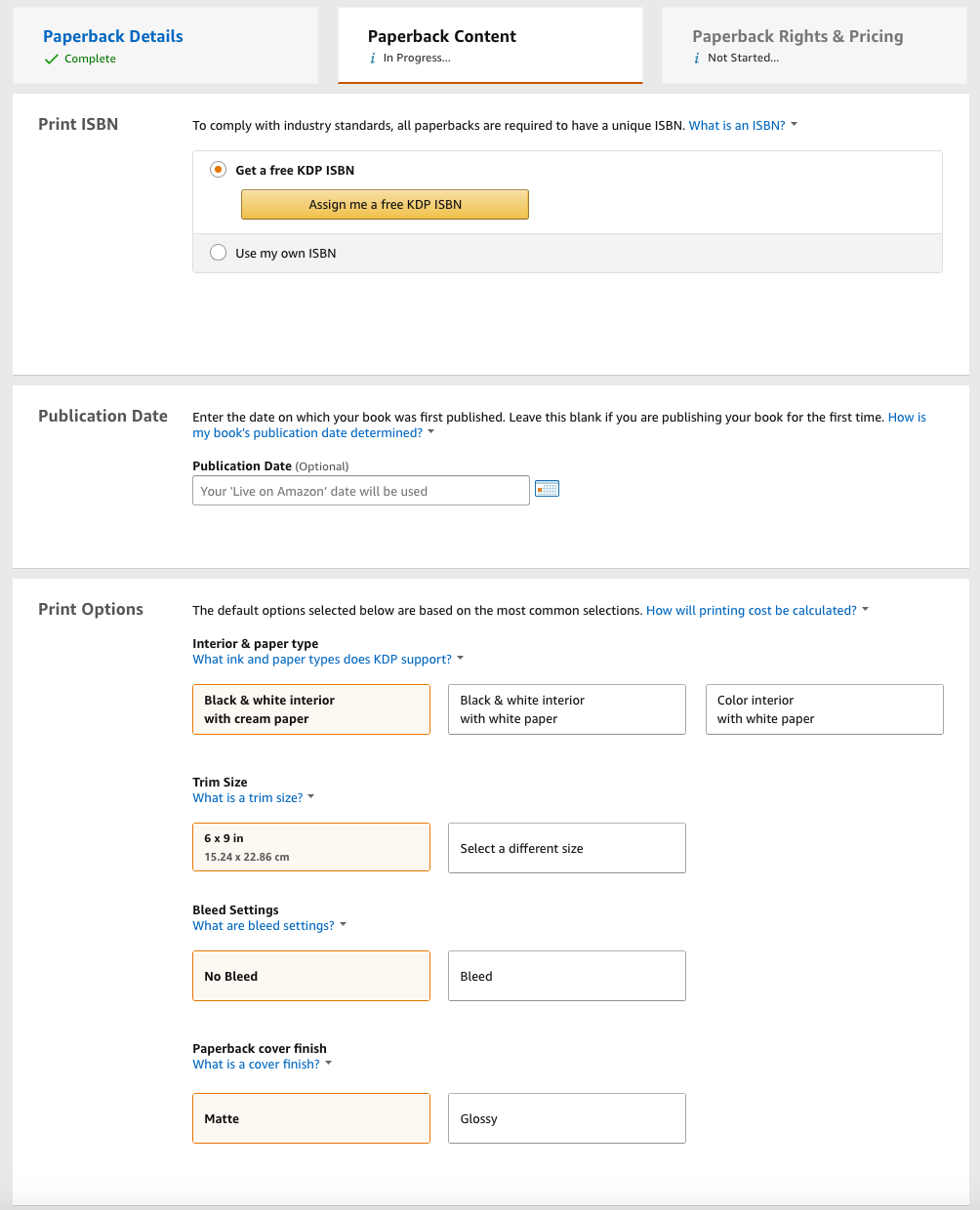In the displayed image, we see a detailed workflow page from a self-publishing platform, featuring various clickable buttons and options for completing the book setup process. 

At the top of the page, there is a section labeled "Paperback Details" with a check mark indicating it is complete. To the right of this section is another labeled "Paperback Content," marked as "In Progress." Adjacent to these sections, there is a grayed-out box titled "Paperback Rights and Pricing," suggesting it is the next step in the process.

The main section focused on the screen is the "Paperback Content." At the top, there is a heading "Print ISBN," accompanied by a note explaining that all paperbacks must have a unique ISBN to comply with industry standards. Below this note, there is a toggle option to "Get a free KDP-ISBN," along with an alternative option to use your own ISBN.

Further down, there is a section for the "Publication Date" with instructions to enter the date the book was first published, or to leave this field blank if publishing for the first time. An area is provided for entering the publication date.

At the bottom of the screen, we see the "Print Options" heading with a note that the default selections are based on the most common choices. This includes:

- "Interior & Paper Type": Currently set to "Black and White Interior with Cream Paper."
- "Trim Size": Displayed as "6 x 9 inches."
- "Bleed Settings": Listed as "No Bleed."
- "Paperback Cover Finish": Currently set to "Matte."

Additional options are provided for each section:
- For "Interior & Paper Type," choices include "Black and White Interior with White Paper" and "Color Interior with White Paper."
- For "Trim Size," users can select different dimensions besides the default 6 x 9 inches.
- For "Bleed Settings," the options are "No Bleed" or "Bleed."
- For "Paperback Cover Finish," users can select either "Matte" or "Glossy."

Overall, the image reflects a structured and detailed interface for setting up a paperback book, guiding the user through each step with clear options and instructions.